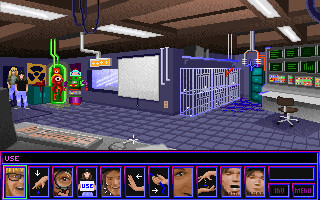The image is a pixelated, retro-style landscape graphic resembling a scene from an old video game, likely from the 80s or 90s. It depicts a lab environment filled with various scientific apparatus and characters. In the foreground, there's a large, light gray desk with multiple monitors displaying green, red, yellow, and blue blocks, reminiscent of old-school green text lines on computer screens, much like those seen on a Commodore 64. Below these monitors, there's a row of colorful screens and a classic desk chair, characterized by its round, metallic frame and sitting atop a small dark blue carpet. 

Behind the desk, to the left, are two rows of six animal cages stacked on top of one another, adjacent to a dark gray wall with pipes and an aquarium. The scene also features a series of filing cabinets in a bluish-green hue and multiple fluorescent lights on the ceiling, which has a mix of light and dark brown panels. Suspended from the ceiling, there are Telsa coil-like metal rings generating a blue lightning bolt. 

A prominent yellow radiation warning sign with black markings is visible, adding to the atmospheric tension. Characters include a green robot, a red tentacle alien in a test tube, and a female figure with long blonde hair. These characters are seen to the left, near the entrance marked by a biohazard symbol. Additionally, a status bar at the bottom of the screen displays portrait-oriented cards with various graphics, indicating it might be a story-based digital game.